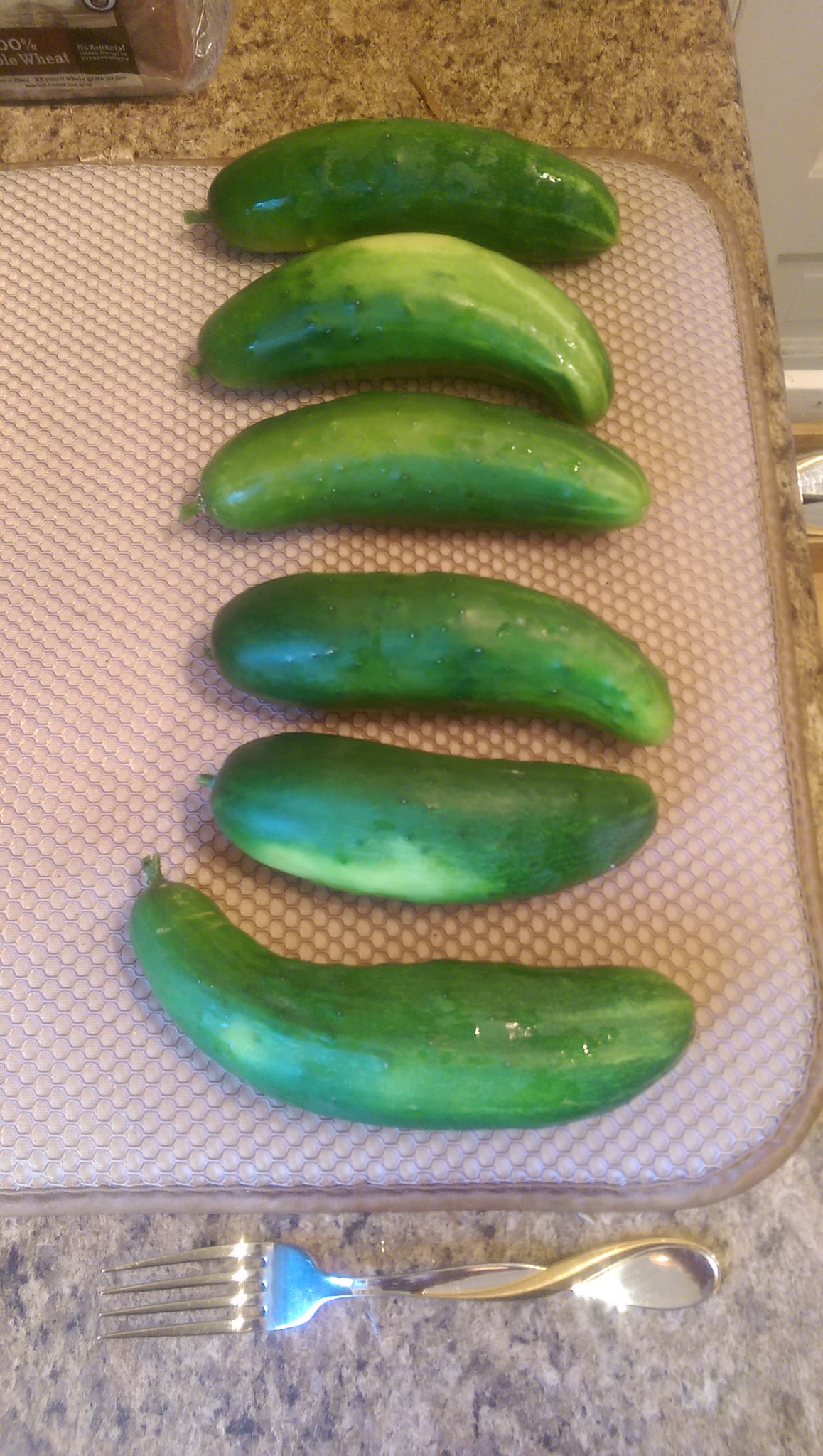This is a detailed color photograph depicting six green cucumbers arranged in a vertical line atop a white drying mat with a woven pattern. The cucumbers exhibit distinct characteristics: three at the top curve downwards, the middle one is straight, and the bottom two curve upwards. Each cucumber varies slightly in shape and coloration, with some displaying light green spots amidst their overall green hue.

Beneath the cucumbers at the bottom of the tray lies a silver fork with an unusual handle that twists into an infinity symbol. Light reflects off the end of the fork, drawing attention to its intricate design. The mat is placed on a counter that appears to be either marble or a light beige Formica with a darker grey mottling pattern, which adds texture to the scene.

In the top left corner of the photograph, a square wooden object with indistinct white writing is partially visible. The upper right corner shows a backdrop of indistinct greyness with potential bands of light, adding depth to the composition.